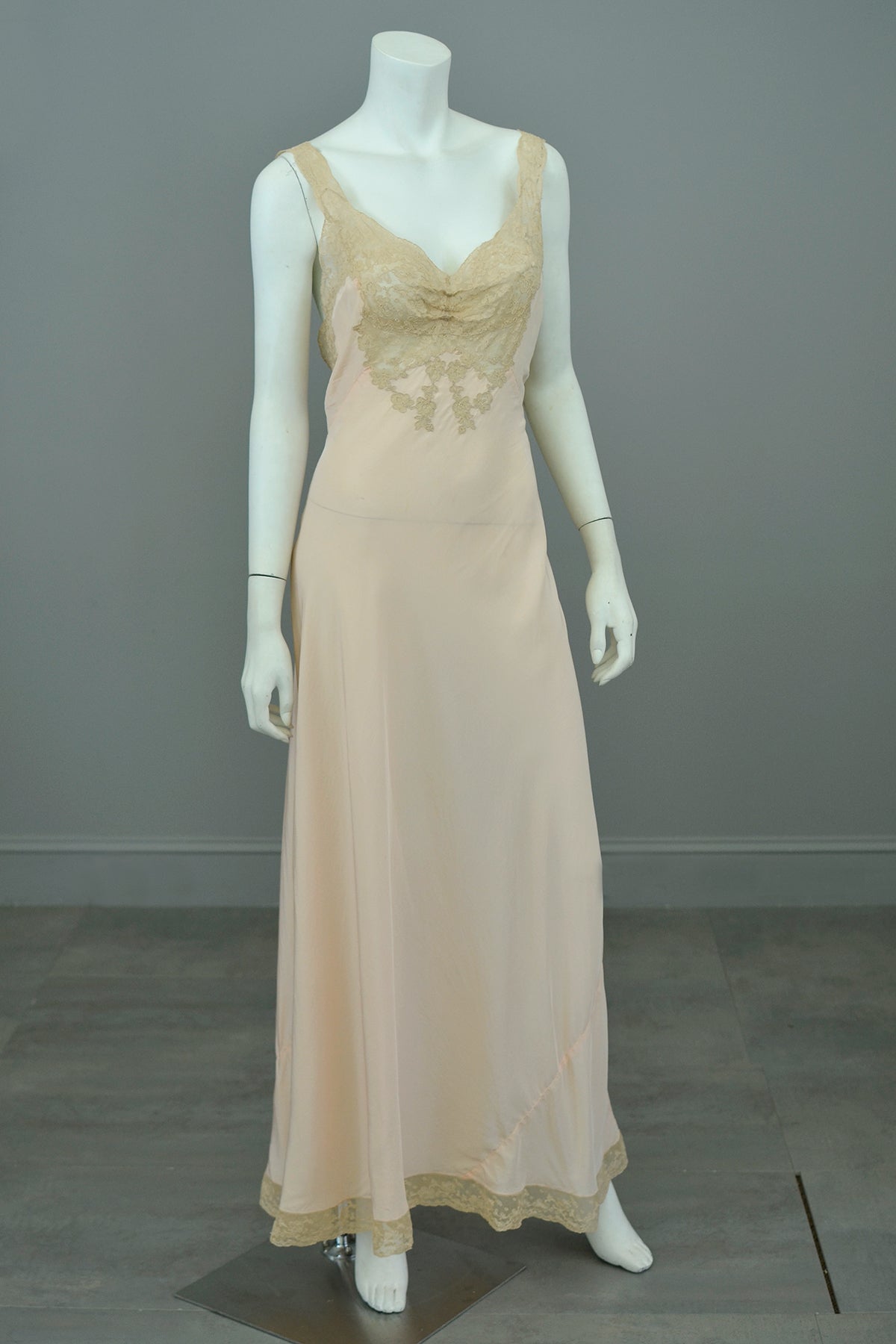This indoor photograph captures a detailed and aesthetically pleasing scene centered on a white, headless mannequin. The mannequin, standing on a light gray and brown wood-paneled floor, is adorned in a long, peach-colored nightgown that reaches down to the ankles. This vintage-style piece of lingerie features delicate lace straps that extend over the shoulders, forming an intricate bodice. The lace, a slightly darker peach, continues as a fringe at the hem of the nightgown. The fabric itself appears to be light and sheer, possibly made of silk or a similar material, adding a flowy, ethereal quality to the garment. The entire setup is set against a simple gray wall, emphasizing the elegance of the nightgown. The photograph, slightly blurry in some parts, captures the subtle details and textures of both the mannequin and the nightgown, creating an understated yet captivating image.